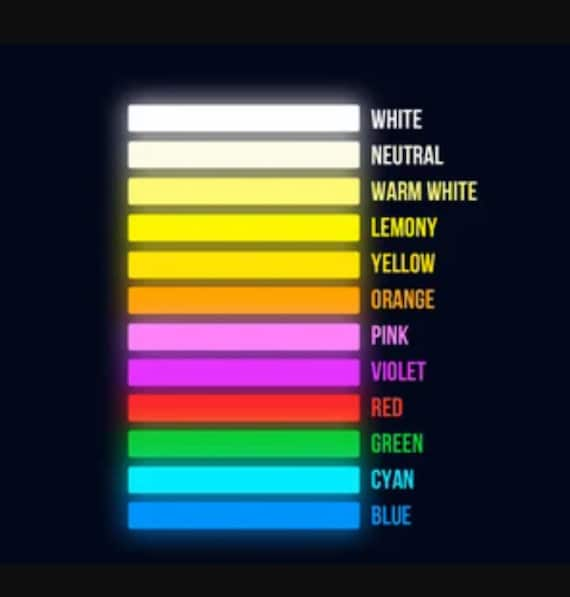This image is a brightly colored LED color chart, presenting a range of vibrant hues against a black background. The chart starts with white and continues through neutral, warm white, lemony, yellow, orange, pink, violet, red, green, cyan, and blue. Each color is represented by a glowing, fluorescent strip alongside its name, forming a vertical, long rectangular bar. The color names are listed on the right side of each corresponding strip. The detailed color gradient shines vividly, displaying the varied temperatures and hues in which an LED light bulb can illuminate. The chart has dark blue borders at the top and bottom. For further details, visit www.FEMA.gov.